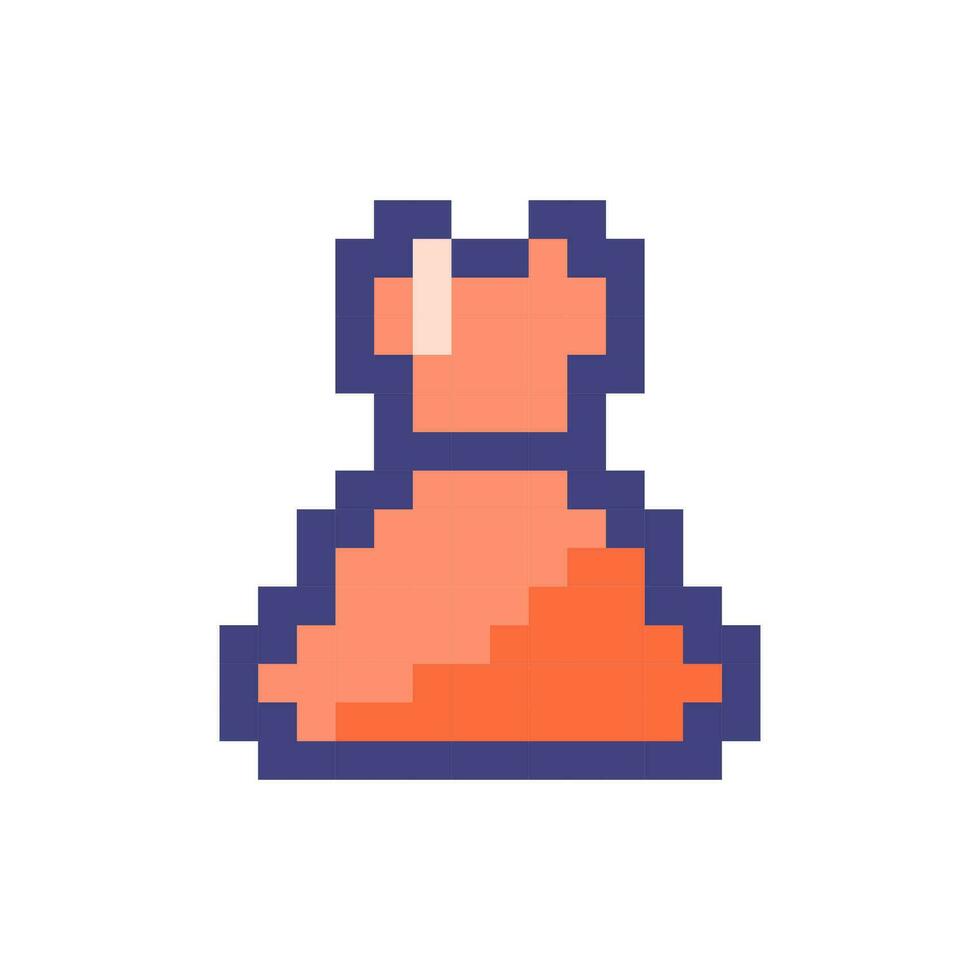This image features a digitally created 8-bit art piece centered on a white background. The object depicted resembles an old arcade game graphic, possibly a potion bottle or vase, rendered in a combination of orange and blue hues. The lower part of this object has a rounded triangular shape encased in blue lines, with the bottom right segment in dark orange and the upper left in pale orange. The upper section features additional pale orange areas and a distinct rectangular off-white highlight, suggesting a light reflection. The entire creation is framed by dark blue, dark purple, and coral-colored outlines, adding contrast and definition. Rising vertically from the base, there is a slender white line, seemingly unfinished or uncolored, contributing to the overall retro, pixelated aesthetic that hints at a simpler, yet nostalgic, digital era.